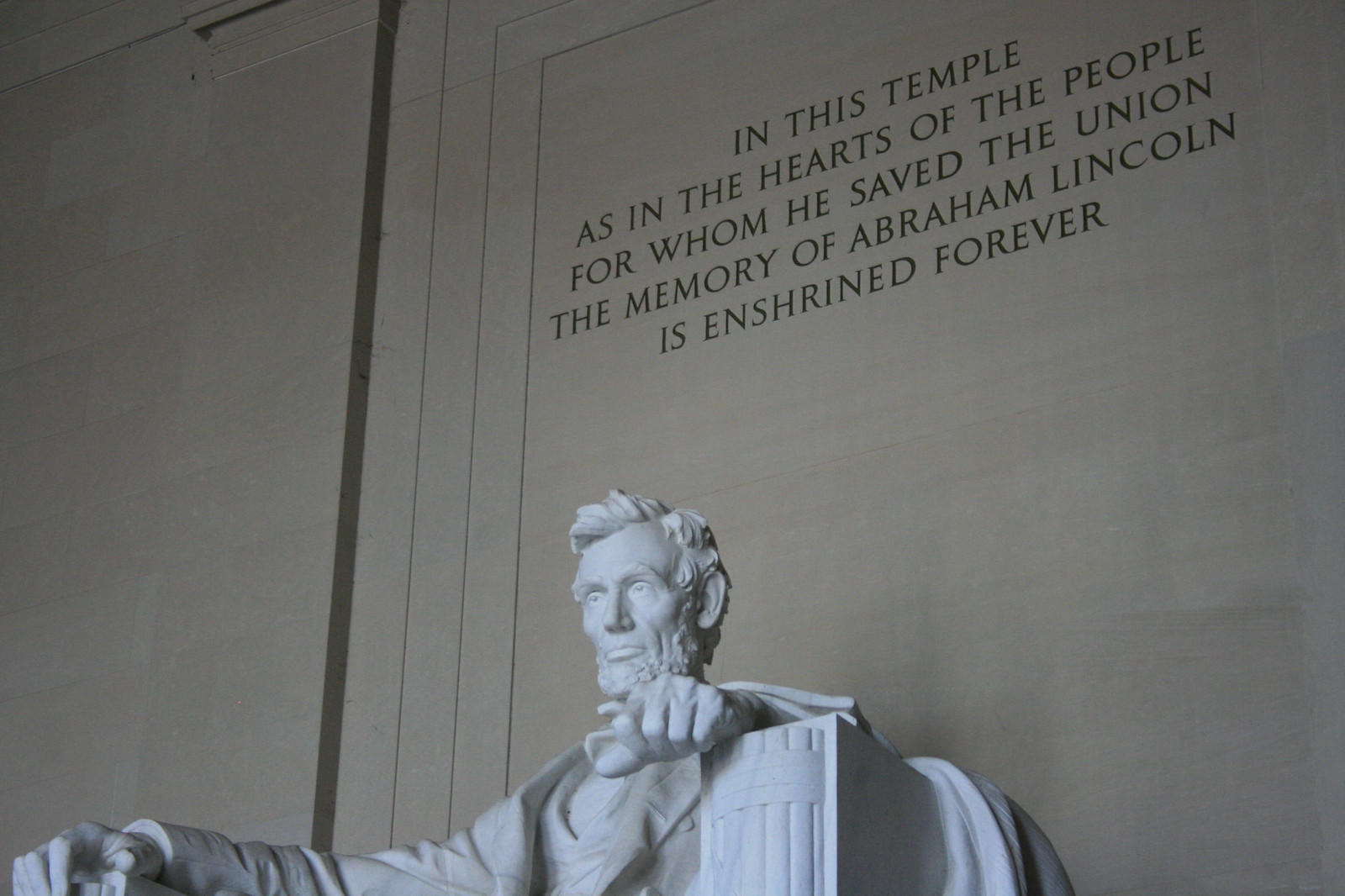The image depicts the iconic Abraham Lincoln statue at the Lincoln Memorial in Washington D.C. Captured from an angled perspective on the lower right side, the photograph highlights Lincoln seated in his chair, with his body slightly leftward and mostly showing his upper torso and resting arms. The statue stands out in a striking milky white against the contrasting beige stone wall behind it. The inscription above Lincoln’s head reads in uppercase black lettering: "IN THIS TEMPLE, AS IN THE HEARTS OF THE PEOPLE FOR WHOM HE SAVED THE UNION, THE MEMORY OF ABRAHAM LINCOLN IS ENSHRINED FOREVER." The wall itself has a tan, layered appearance, adding depth to the background. Lincoln’s distinctive features, including his prominent nose, abundant hair, and signature beard, are clearly visible as he gazes thoughtfully into the distance.